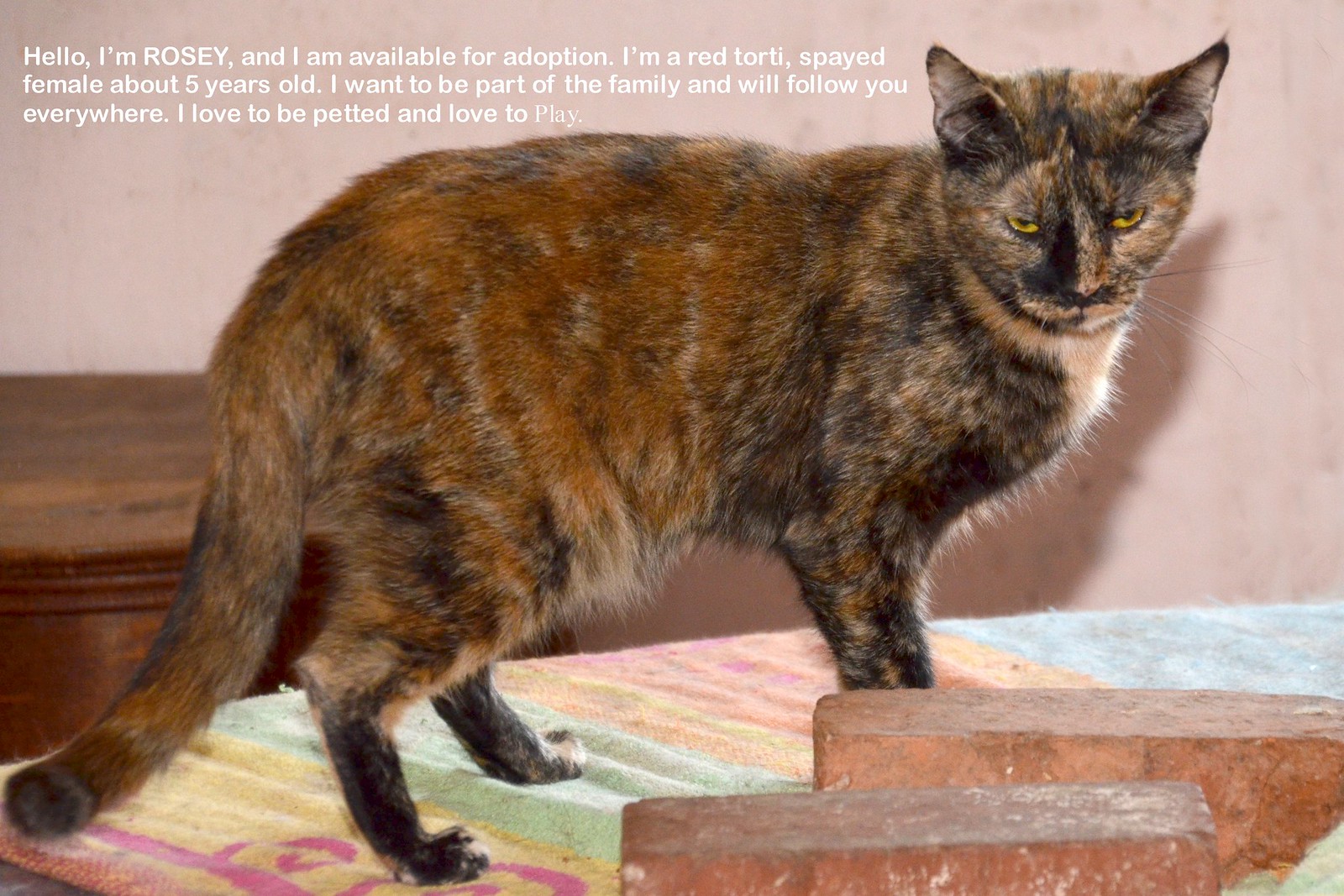In the image, a beautiful tortoiseshell cat named Rosie is standing on a multicolored beach towel laid on a table. Rosie's fur features a striking mix of black, orange, brown, and light beige, giving her a Halloween-like appearance, with a face that is partially black and partially orange. She has bright yellow eyes that look slightly downward towards the camera, creating a gentle, glowering expression. The cat's body is facing to the right while her head is turned towards us, highlighting her soft and thick fur. 

In the foreground, there are two red bricks placed on the right side of the table, adding a curious touch to the scene. Behind Rosie, the background consists of a pink-colored wall and a brown wooden dresser to the left. Additional white text at the top left of the image reads, "Hello, I'm Rosie, and I am available for adoption. I'm a red Tortie, spayed female, about five years old. I want to be part of the family and will follow you everywhere. I love to be petted and love to play." The lighting casts a soft glow on Rosie and her surroundings, emphasizing the sheen of her fur and creating a shadow on the pink wall.